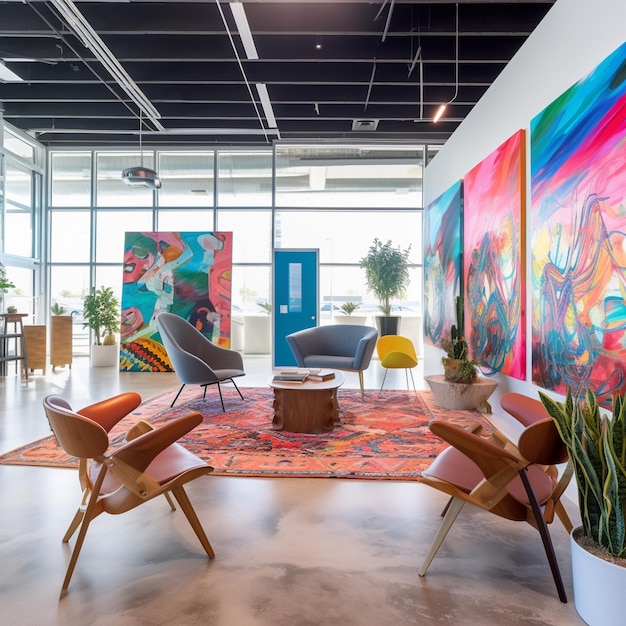This image captures a bright, open-concept space that suggests a modern art gallery or a chic office setting. The room features expansive glass windows on the back wall, divided into squares, allowing ample natural light to flood in, and possibly indicates a storefront or gallery facing a road. The left wall also appears to be made of windows, enhancing the airy feel of the space. The industrial-style ceiling is characterized by dark metal panels with several hanging light fixtures. 

Dominating the right wall are three large, vibrant abstract paintings composed of colorful stripes and swooshes, mainly in pink and blue hues. Complementing these, an additional abstract painting in a similar color palette leans against the back wall of windows. The room's concrete floor is softened by a large, intricate rug placed centrally.

Furnishing the space are two artistically designed wooden chairs with tannish-red leather seats in the foreground, a substantial wooden table surrounded by two more wooden chairs, a yellow chair with metal legs, and two gray chairs positioned towards the back. A blue door adds another splash of color to the back wall, enhancing the modern aesthetic of the setting. This well-lit room, with its artistic decorations and contemporary furniture, vividly conveys the atmosphere of a stylish gallery or office space.